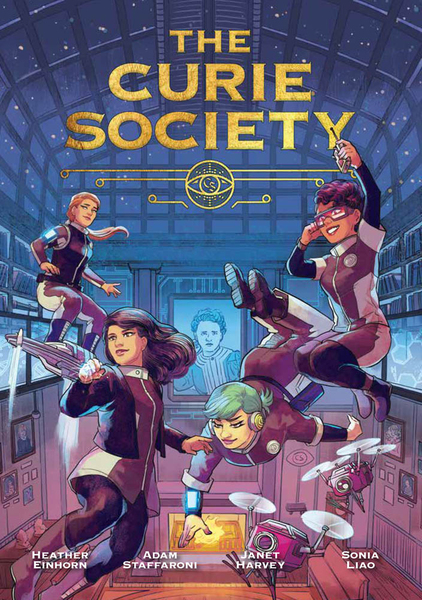This detailed illustration is the front cover of what appears to be a comic book titled "The Curie Society," rendered in a vibrant, cartoonish anime style. The cover features four female figures, each wearing distinctive uniforms in a color scheme of purple and light violet, seemingly floating or flying in mid-air, hinting at possible anti-gravity or flight abilities as their superpower. These characters share the space with a pair of pink, bird-footed drone cameras equipped with propellers and camera lenses.

At the top of the cover, the title "The Curie Society" is prominently displayed in large, gold lettering. Below, in smaller white text, the names of the creators are listed: Heather Einhorn, Adam Staffaroni, Janet Harvey, and Sonia Liao.

The scene is set within a room characterized by its purple walls and a large, transparent glass ceiling revealing a dark blue night sky filled with stars. The lower section of the room includes various details like seating areas, a fireplace, bookshelves, and a screen TV. In the background, a faint portrait of a woman, likely representing Marie Curie and aligning with the title, adds a historical touch to the futuristic setting, blending elements of past and present.